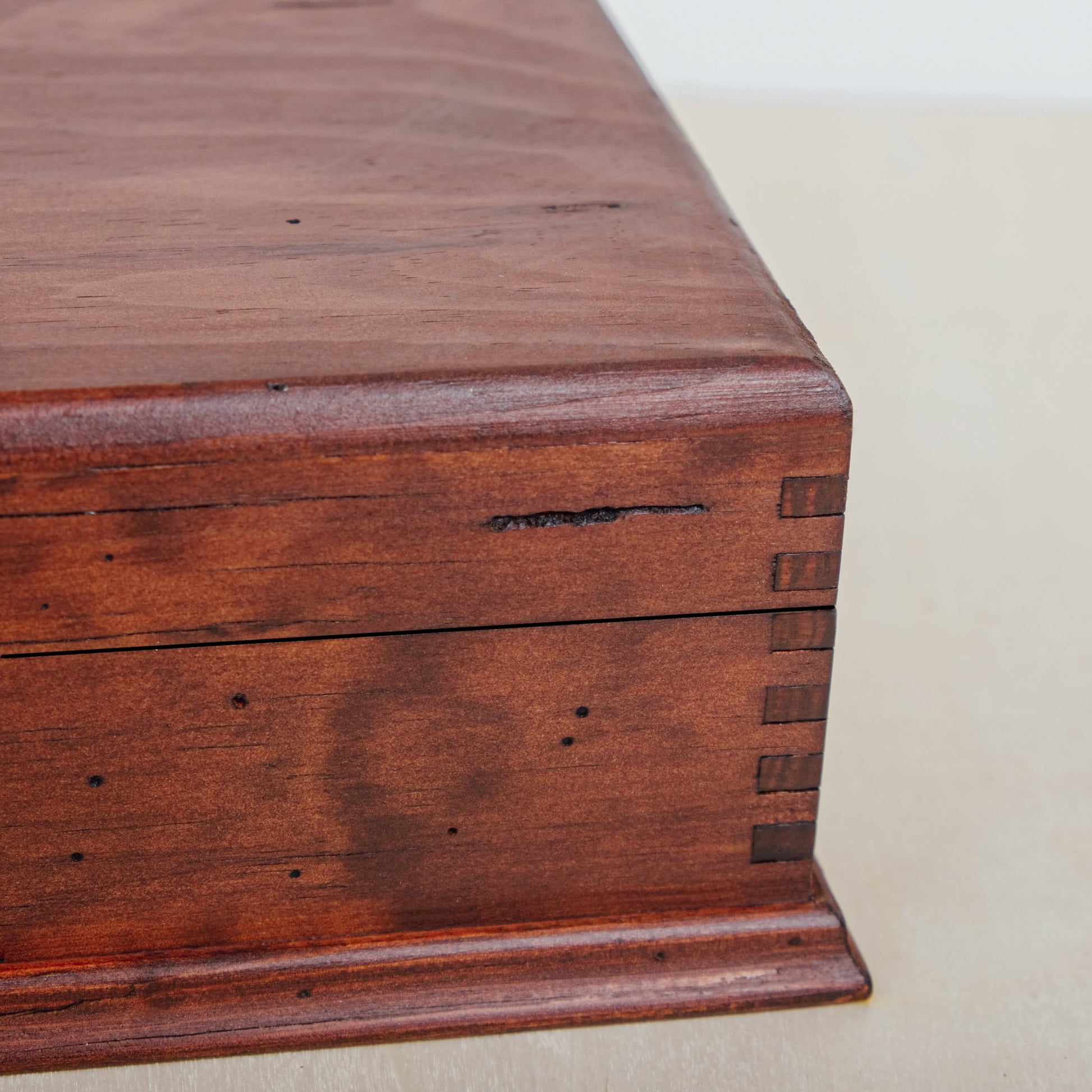The image depicts the corner of a brown, wooden object with a rectangular, solid form, featuring detailed grain and a stained brown finish. The wooden item is photographed on a flat, white background, emphasized by the clean and simple contrast. The upper left and lower left corners, as well as the center, are visible in the image, with the rest of the object extending out of the frame. This object includes a beveled border along its bottom edge, giving it a defined lip. It appears to have been intricately constructed with interlocking joints resembling a puzzle, indicative of a well-crafted box or container. The visible corner displays the precise positioning of the edges and the beveled detail suggests thoughtful craftsmanship. Despite its limited visibility, the combination of the grain, staining, and beveled bottom suggests the object could be a wooden box or even a step, featuring a composition that balances functionality with aesthetic craftsmanship.